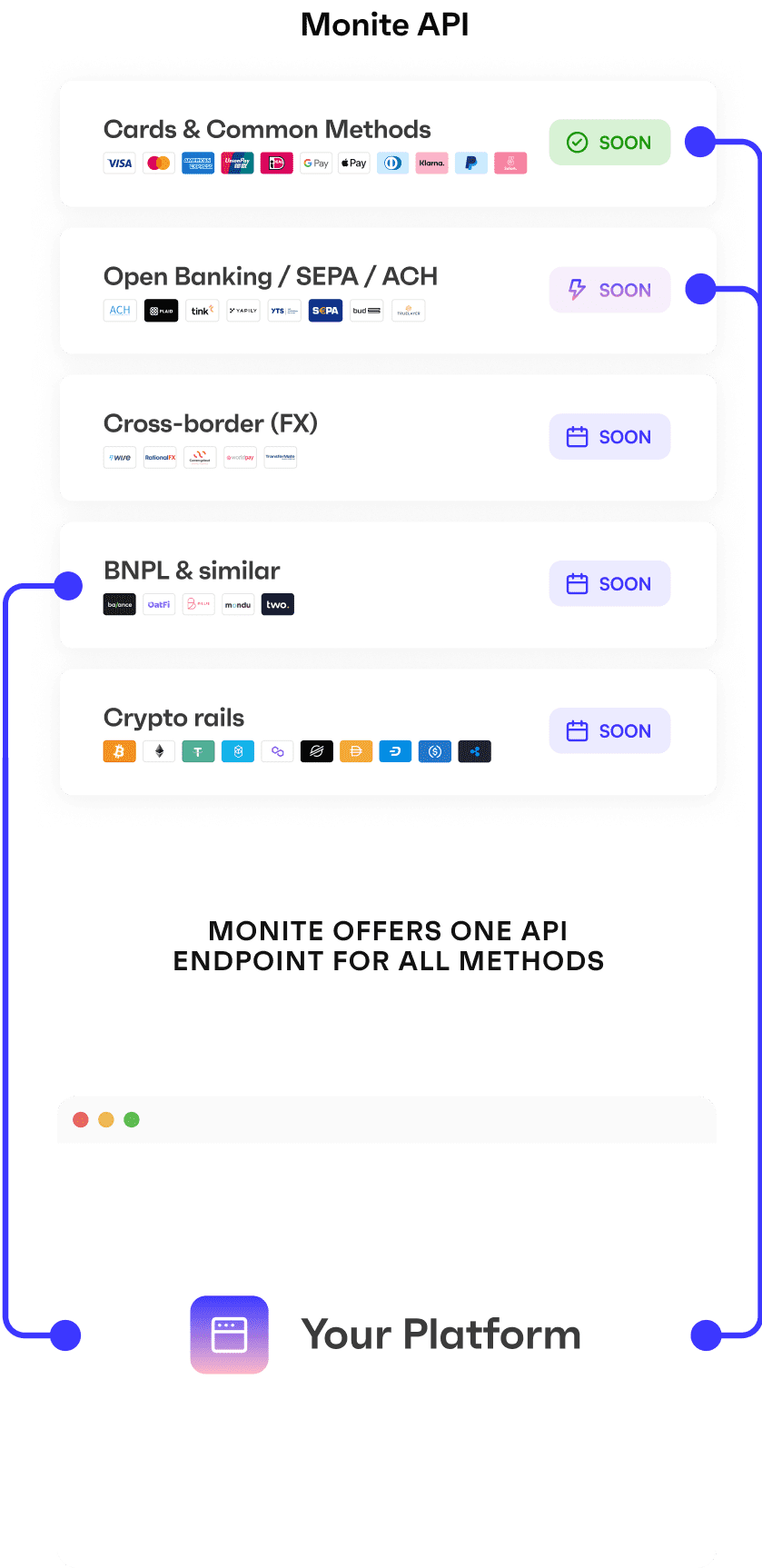This image showcases the Monite API platform, visually represented through a series of interconnected cards. The cards, which are vibrantly colored, represent various categories such as Banking, Cards, Common Methods, and Open Banking. Prominently, some of these cards are marked with "Coming Soon," indicating upcoming features or integrations. The layout leads to a centralized platform, suggesting a comprehensive solution for cross-border transactions and crypto rails. The user interface is visually rich, incorporating dynamic elements like purple lines and circular dots, though their exact function remains unclear. Overall, the image appears to illustrate Monite API's extensive and evolving financial technology offerings.